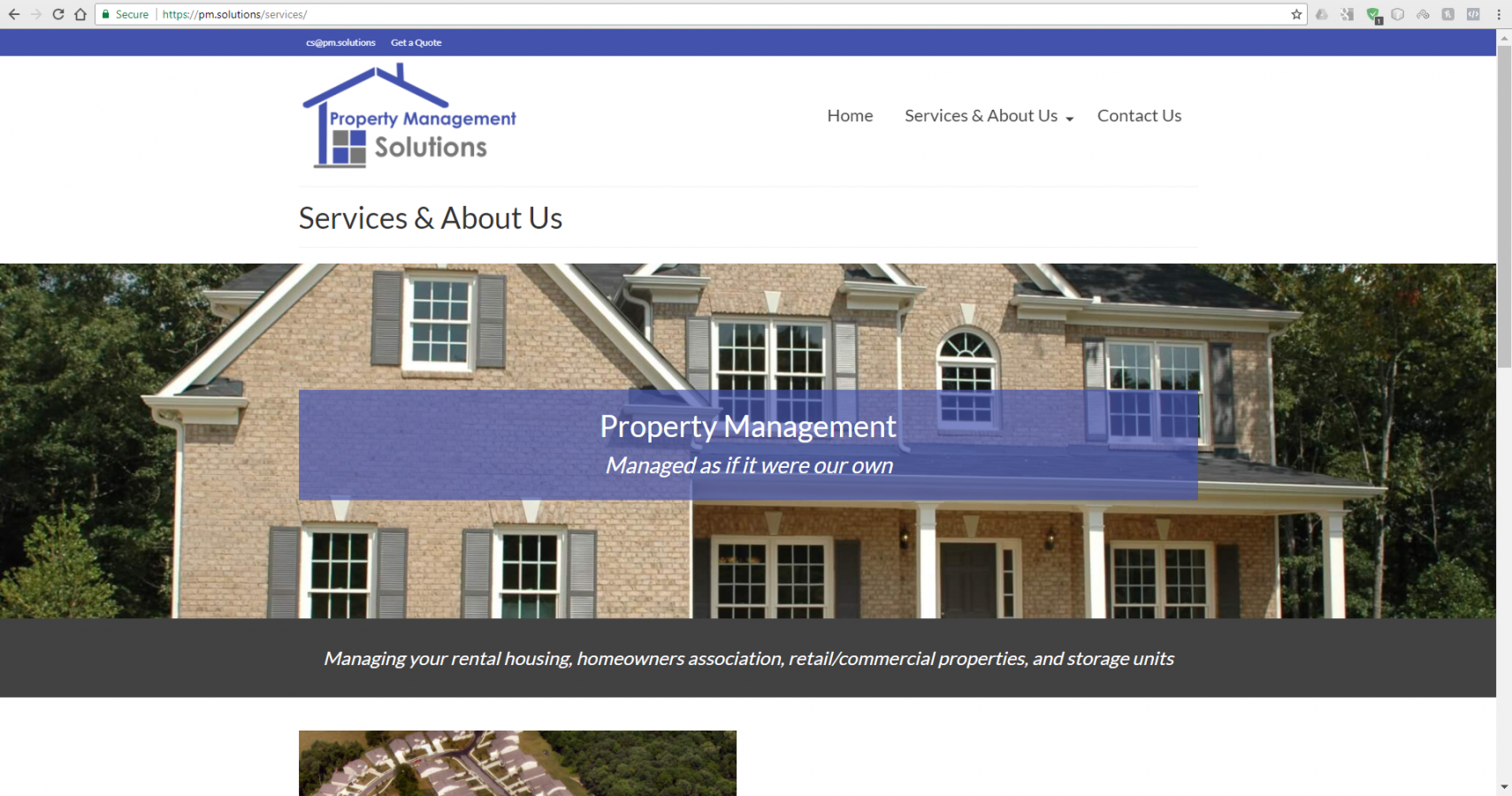The image features a detailed logo for a property management company set against a blue rectangular background. The logo itself depicts a stylized house with four shaded squares in gray-blue and blue-gray tones. Surrounding the house are lush green trees and a subtle glimpse of the sky, creating a serene and inviting atmosphere.

The header section of the image prominently displays the company's services, which include:

- Property Management Solutions
- Home Services
- About Us
- Contact Us

Additionally, there's a button labeled "Get a Quote."

At the bottom of the image, there is a gray rectangular banner with text that reads, "Managing your rental housing, homeowners association, retail/commercial properties, and storage units."

The image also includes a neighborhood scene, captured from a slightly elevated, top-down perspective, offering a comprehensive view of the managed properties within a well-maintained community.

Overall, the caption conveys both the aesthetic and the professional services provided by the property management company, using the detailed visual cues from the image.